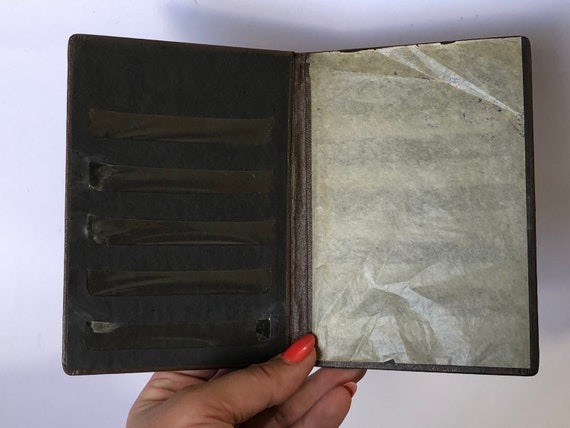In the photograph, a hand with long nails painted in a shade that appears to be orange-red, though it could be interpreted as red, delicately holds what seems to be an old, weathered diary against a light blue background. The skin of the hand is dark-toned, suggesting it might belong to a female. The diary has dark brown leather covers that appear black in certain areas, particularly on the left side, which also features five thin stripes reminiscent of black tape or labels. There are tiny holes on this side, possibly intended for holding small items. On the right, a brittle and crumpled translucent page, through which faint black lines are visible, is draped over the leather cover. The diary casts a shadow against the background, accentuating its aged and mysterious appearance.